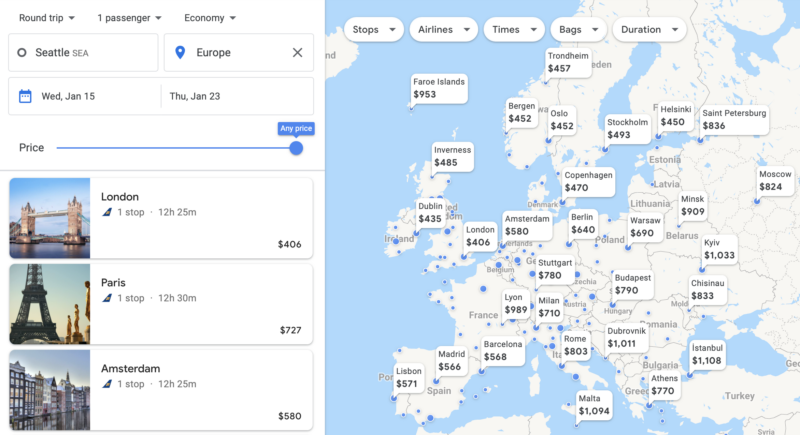The image prominently features a large map oriented to the right side, where various international destinations are marked. The backdrop of the map is blue, likely representing water bodies. At the top of the image, there are tabs labeled: "Stops," "Airlines," "Times," "Bags," and "Duration," which serve as filters for selecting travel preferences.

Each marked destination on the map includes a corresponding number indicating the airfare price. For instance, Copenhagen is at $470, Dublin at $435, Barcelona at $568, Moscow at $824, Rome at $803, Athens at $770, Madrid at $566, Leipzig at $571, Stockholm at $493, London at $406, and Amsterdam at $580. 

On the left side of the image, there's a user interface section designed for booking flights. This area features a form with an initial rectangular input for the departure location and another for the destination. Displayed travel dates are from Wednesday, January 15th, through Thursday, January 23rd, and the price range is set to any amount. Below the booking form, there are quick-select options for popular destinations, including London, Paris (with an Eiffel Tower icon beside it), and Amsterdam, listed at $580.